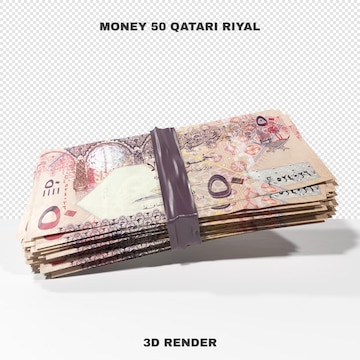The image shows a realistic 3D rendering of a stack of Qatari Riyal banknotes, each with intricate design features. The stack is secured with a black ribbon or band, resembling duct tape, and the individual bills are a shade of brown with black, darker brown, red, and pink markings. The top right corner of the image has the text "Money 50 Qatari Riyal" written in black ink, signifying the currency type and denomination. The bottom half of the image displays the text "3D Render" also in black ink, indicating that the image is a digital creation. The notes bear complex illustrations, potentially including architectural elements such as arches, though the design details are somewhat indistinct. The background is a combination of white at the bottom, where the stack casts a shadow, and a checkered pattern at the top, implying the background has been digitally removed.